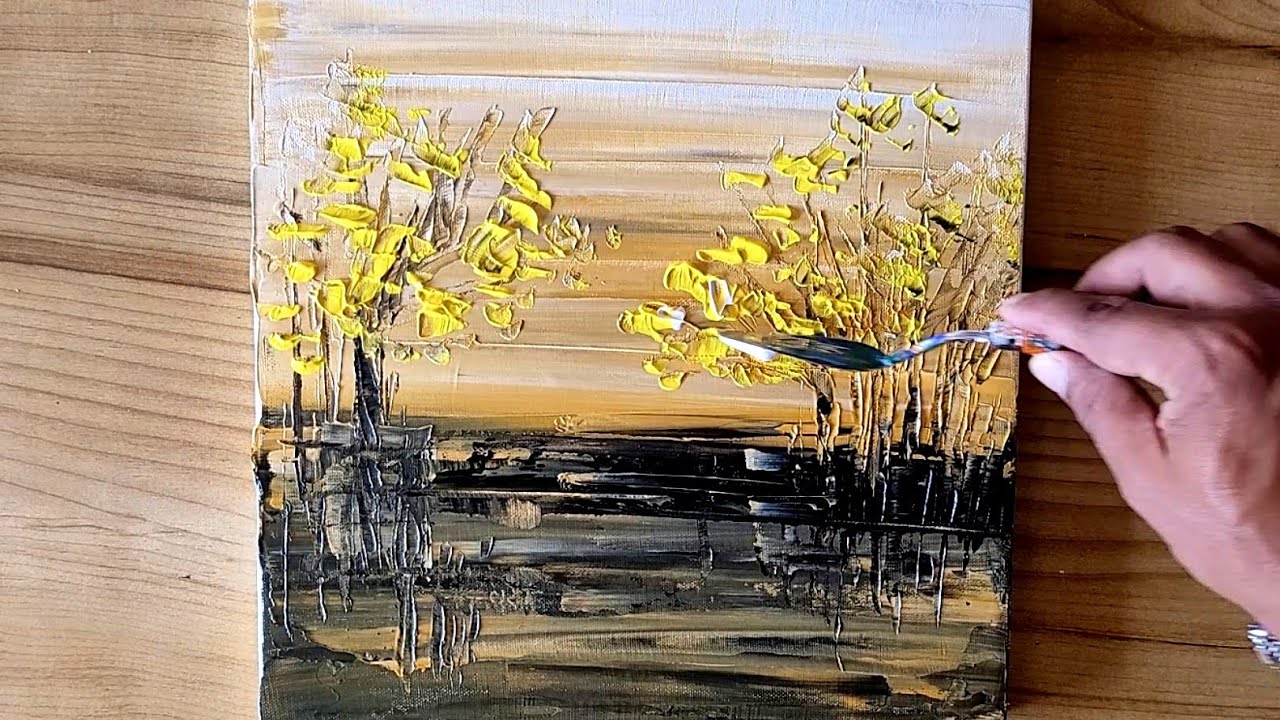The photograph captures a detailed scene of a painter mid-process, focusing on their work from a close-up perspective. The artist, potentially male, is seen using their right hand to hold a paintbrush between their thumb, pointer, and possibly middle fingers. The hand appears to be either African-American, Hispanic, or simply tan-skinned, but the specifics are unclear. The subject of the painting is a nature scene, primarily featuring sparse, yellow leaves on what seem to be trees. The upper part of the canvas showcases a hazy sky blending orange, white, and cream colors, while the bottom simulates a water body with reflective black and gray swirls.

The painting, unfinished, includes some additional intricate details such as brown stripes across the upper part and hints of white, possibly depicting the sky or tree trunks. Yellow flowers are also being highlighted with white paint, particularly on the right side of the canvas. The scene implies a serene, possibly swampy environment. The canvas itself is positioned on a medium-brown wooden table, with horizontal wood grain clearly visible, providing a rustic backdrop that enhances the artistic atmosphere. The paintbrush in the artist's hand is actively engaged in adding white details to the yellow flowers, creating a dynamic snapshot of the creative process.